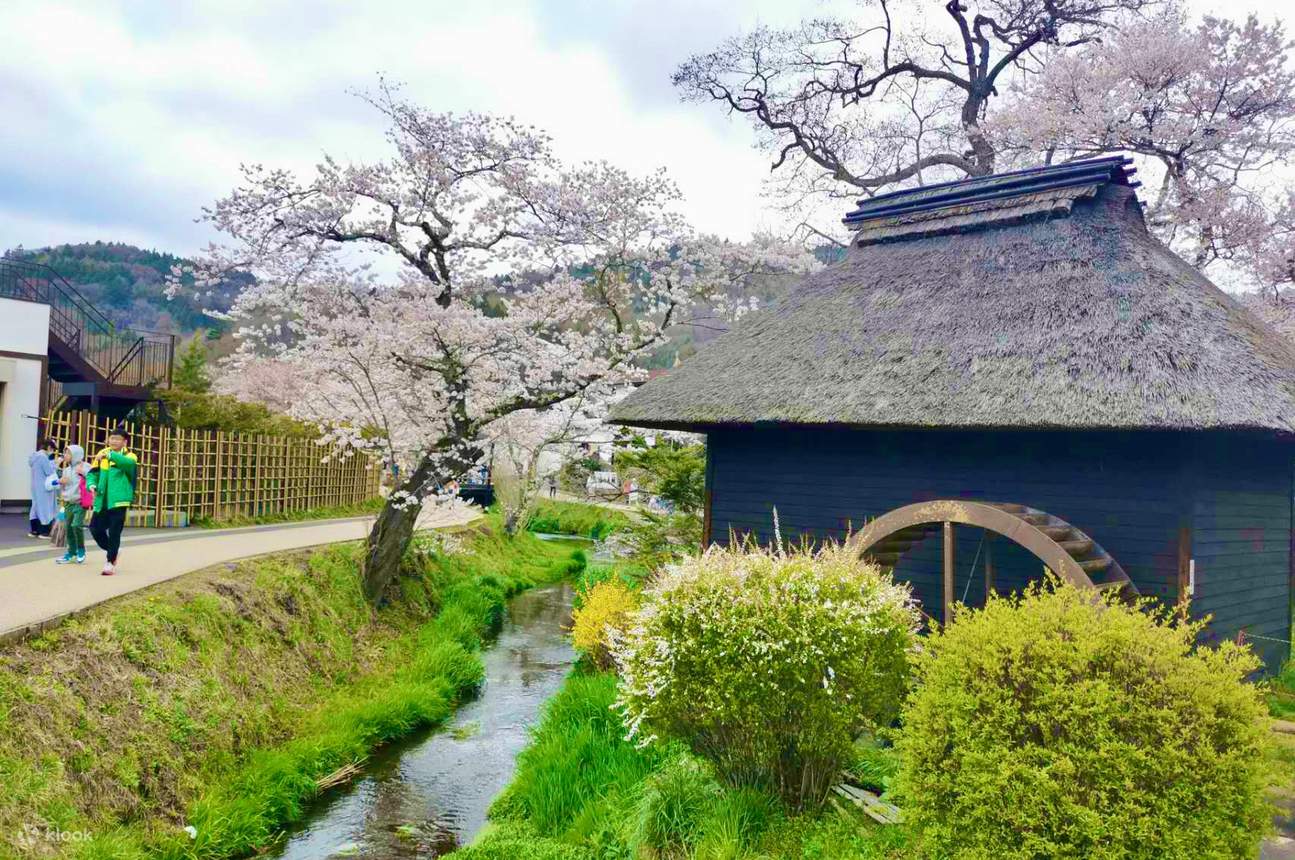The full-color photograph, captured outdoors on a cloudy day with natural light, showcases a picturesque scene reminiscent of a rural area in Japan. It is a square image predominantly composed of an overcast sky with scattered clouds and hints of blue peeking through in the top left. Below, and extending to the upper right corner, fruit trees draped in delicate white blossoms—likely cherry blossoms—create a serene, floral canopy.

Dominating the center right is a quaint blue wooden building adorned with a thatched roof. This structure, seemingly a water mill, features a rustic water wheel framed by a couple of flourishing bushes. Below, a small stream winds its way vertically up from the bottom of the image, paralleled by a walking path bustling with activity. Three figures stroll along this path; notably, one individual in a green and yellow jacket advances forward, while another, cloaked in a hooded garment, has paused for an unknown reason. In the distance, behind the main scene, the silhouette of mountainous terrain rises gently, completing the tranquil, layered composition of this idyllic landscape.